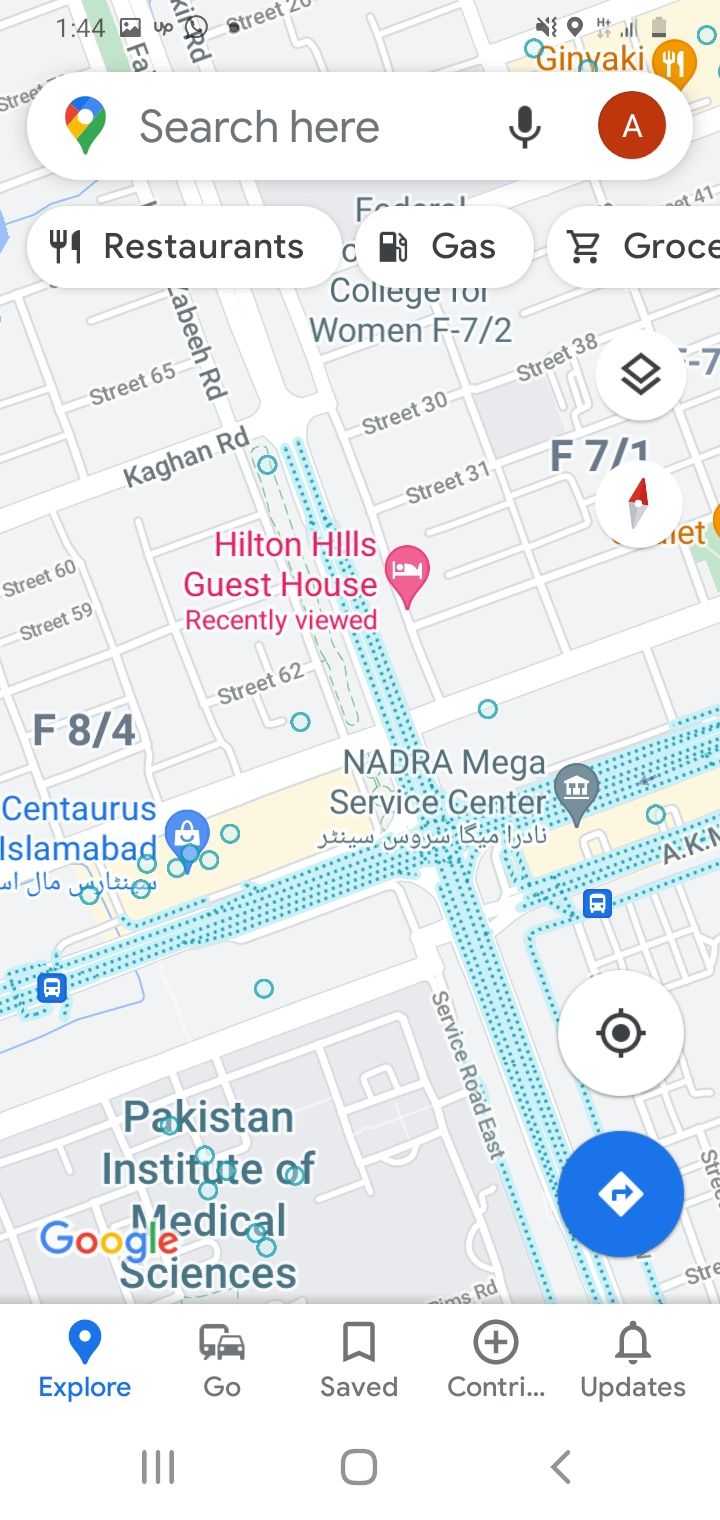Caption: 

The image displays a map interface with a notable search bar at the top which includes a Google search icon, a microphone icon, and the letter "A" enclosed in a circle. Below the search bar, there are options for "Restaurants," "Gas," and "Groceries," though the word "Groceries" is partially cut off. The map itself occupies the majority of the image, featuring streets highlighted in turquoise against a backdrop of white streets and gray land areas. Yellow patches sporadically appear, indicating specific locations of interest.

Several points of interest are prominently marked on the map, including a pink marker for "Hilton Hills Guest House" which has been recently viewed, and a blue marker for "Centris, Taurus, Islamabad." Another highlighted location at the bottom of the map is the "Pakistan Institute of Medical Science."

The interface includes navigation tools, such as a circle containing another black circle with a compass and an 'X' marked on the edges, signifying possible directions or waypoint tools. Below these navigation tools are categories like "Explore," "Go," "Saved," and an abbreviation "C-O-N-T-R" followed by an ellipsis, and an "Updates" section with a bell icon next to it. The text for "Explore" is in blue, indicating it is currently selected, while the rest are in gray.

Blue dots are scattered across the roads, though their specific purpose is unclear. The map seems to be focused on a location within Pakistan.